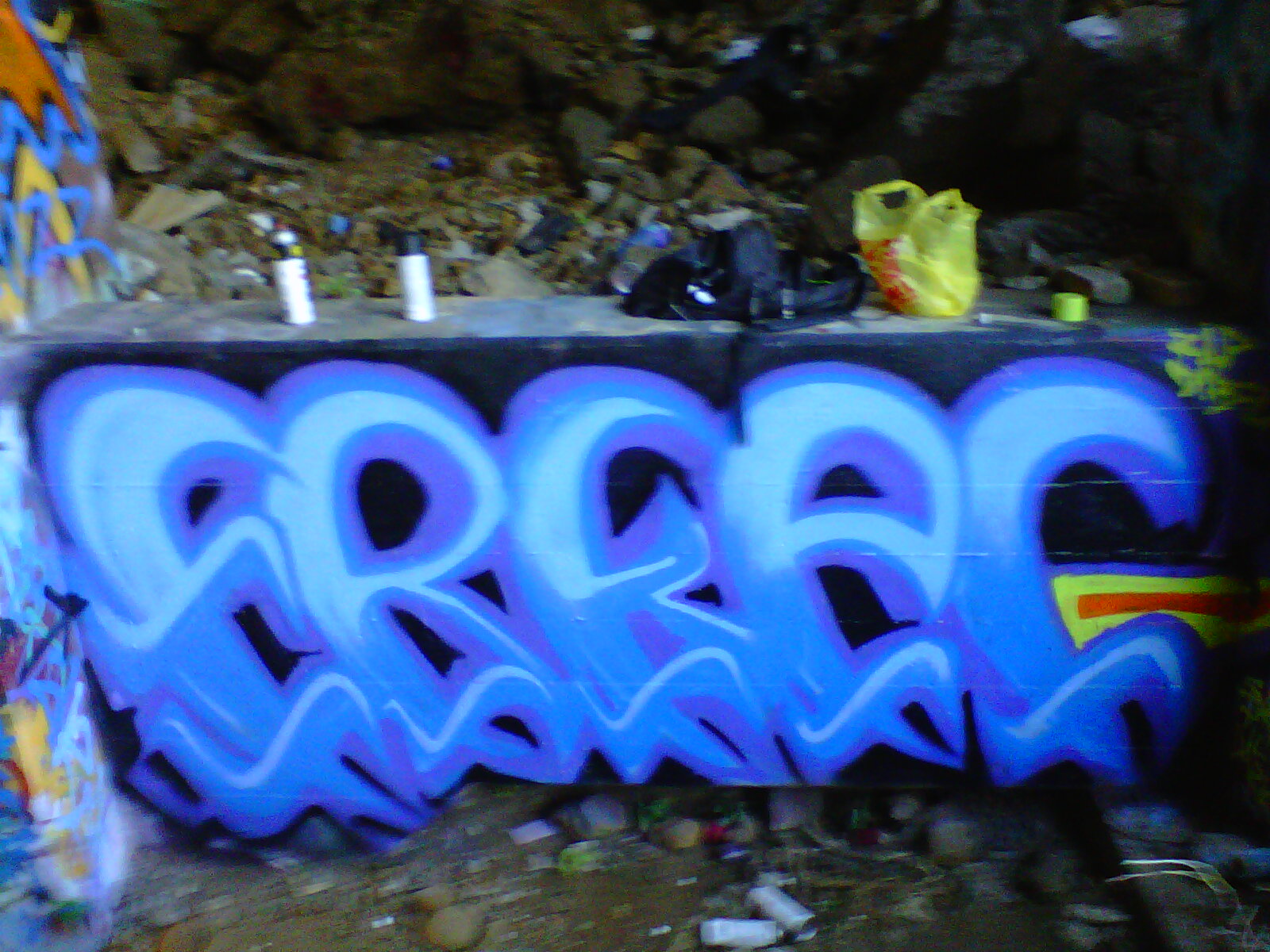The photograph showcases an outdoor graffiti scene on a cement wall, possibly under a bridge or overpass. The graffiti features large, purple lettering that seems to spell out "F-R-E-E-C" or "freak," though the exact words are somewhat indistinguishable. The wall has a black background with dark blue and light blue outlines, accented by yellows and reds. The scene is cluttered with various debris including garbage cans, rocks, a yellow plastic bag, and a black backpack, which might contain the artist's tools. Atop the wall, there are several spray paint cans and a yellow spray can cap. The background of the photograph is filled with broken rock formations and more litter, creating an overall chaotic and degraded urban environment.